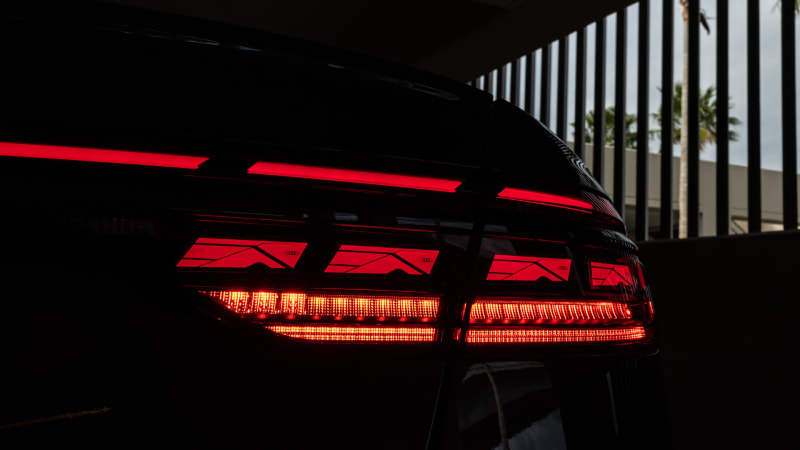This image depicts a car parked in a dimly lit garage, suggesting an indoor or underground setting. The background is quite dark, but slats on the wall let in some light, hinting at a warm climate with visible palm trees and parts of another building beyond. The car, whose specific make and color remain indiscernible due to the darkness, features intricate taillights that are prominently displayed. These taillights consist of three thin, slender red lights at the top, which align with the window's reflection. Below these, three rectangular lights glow, displaying a mix of bright red, reddish-yellow, pink, and intricate patterns of alternating black and bright lights. The scene, accentuated by the variance in colors such as black, gray, white, sky blue, green, and sandy gray, offers a unique and detailed visual of a car in a serene yet somewhat mysterious garage setting.